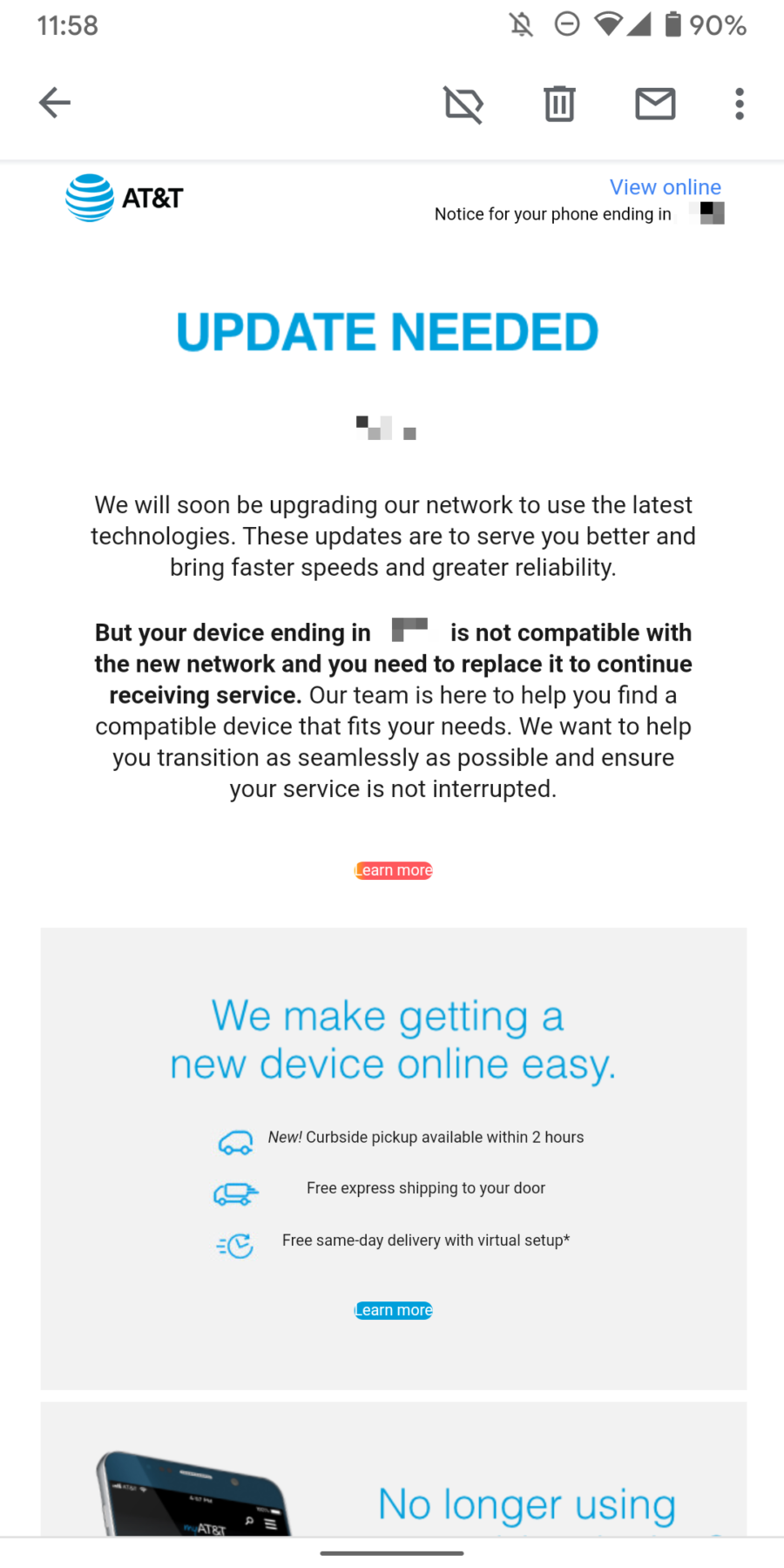The image showcases a smartphone screen displaying a website. The phone's status bar at the top indicates a battery level of 90%, full signal bars, and the current time of 11:58. The carrier appears to be AT&T. 

The website displayed on the phone is an official AT&T page, highlighted with the AT&T logo next to the text. The page prominently features a message in bold blue letters stating, "Update Needed." Below this message, there's a notification that starts with, "Notice for Your Phone Ending In," followed by a shaded-out section likely representing the last digits of the phone number.

A gray, black, and blue icon appears next to a calendar symbol that is marked off. The detailed message further explains that AT&T will soon be upgrading their network to incorporate the latest technologies. It informs the user that these updates aim to provide faster speeds and better reliability. However, the user's current device, indicated by a partially obscured number, is not compatible with the new network. Consequently, the user is advised to replace their device to continue receiving service without interruption.

The page also offers assistance for finding a new compatible device. Emphasis is given to a seamless transition, with assurances that their team is ready to help. 

At the bottom of the notification, there is a red box with white text that reads, "We make getting a new device online easy." This section details various acquisition options, including curbside pickup, free express shipping, and free same-day delivery.

Finally, the lower part of the screen contains a gray box with text explaining the process for no longer using the old phone, accompanied by an image showing the top of a cell phone.